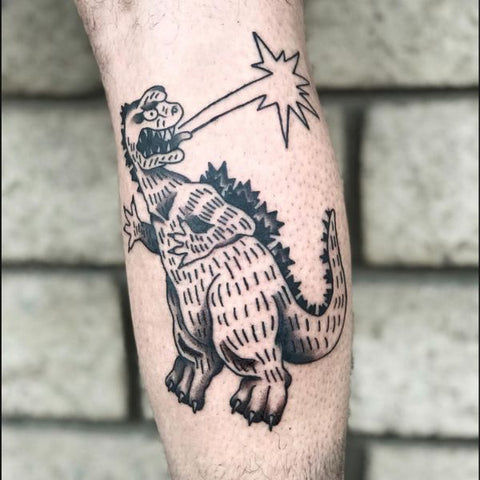This photograph captures a close-up of a partially shaved, hairy white arm, positioned against a light gray brick wall with black mortar joints. The visible section of the arm spans from just above the wrist to just below the elbow. Adorning this area is a black and white tattoo that features a cartoony dragon or possibly a Godzilla-like creature. The dragon, drawn in an animated style, stands upright on its thick hind legs, with a robust tail extending behind. Its spine is adorned with spiky protrusions running down to the tail tip. The creature's head is turned back over its left shoulder, revealing menacing sharp teeth and an open mouth with its tongue sticking out. From its mouth, it appears to be breathing fire or spewing a shooting star, depicted by horizontal lines culminating in a star formation. The dragon's limbs are detailed with three toes and prominent toenails, adding to the whimsical, yet striking nature of the tattoo.